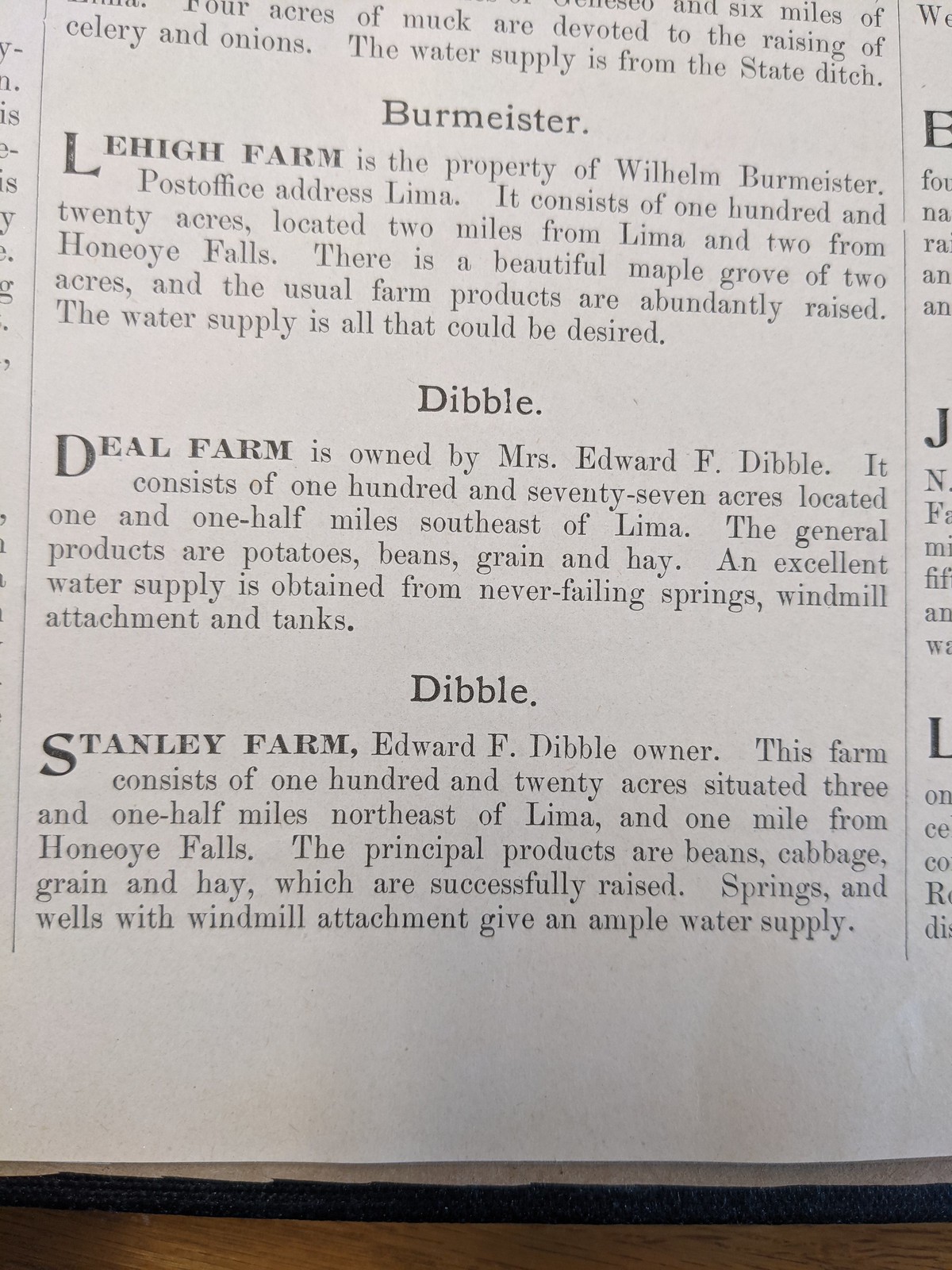The image is an up-close photograph of an off-white newspaper clipping, partially cropped on the left, right, and top edges. It details a publication about three farms, each highlighted in bold black print. The first entry, titled "Burmeister Land Farm," belongs to Wilhelm Burmeister, with a post office address in Lima. This farm spans 120 acres, situated 2 miles from Lima and 2 miles from Honeoye Falls. It boasts a beautiful 2-acre maple grove and a plentiful supply of various farm products. The water supply is described as ideal.

Following that, "Deal Farm," owned by Ms. Edward F. Dibble, encompasses 177 acres and is located 1.5 miles southeast of Lima. It primarily produces potatoes, beans, grains, and hay. The water supply is excellent, sourced from reliable springs with windmill attachments and tanks.

Lastly, "Stanley Farm," owned by Edward F. Dibble, covers 120 acres 3.5 miles northeast of Lima and 1 mile from Honeoye Falls. It successfully raises beans, cabbage, grain, and hay. Like the other farms, it has a robust water supply from springs and wells equipped with windmill attachments. The clipping lies atop a surface with a visible horizontal strip of brown wood at the bottom.